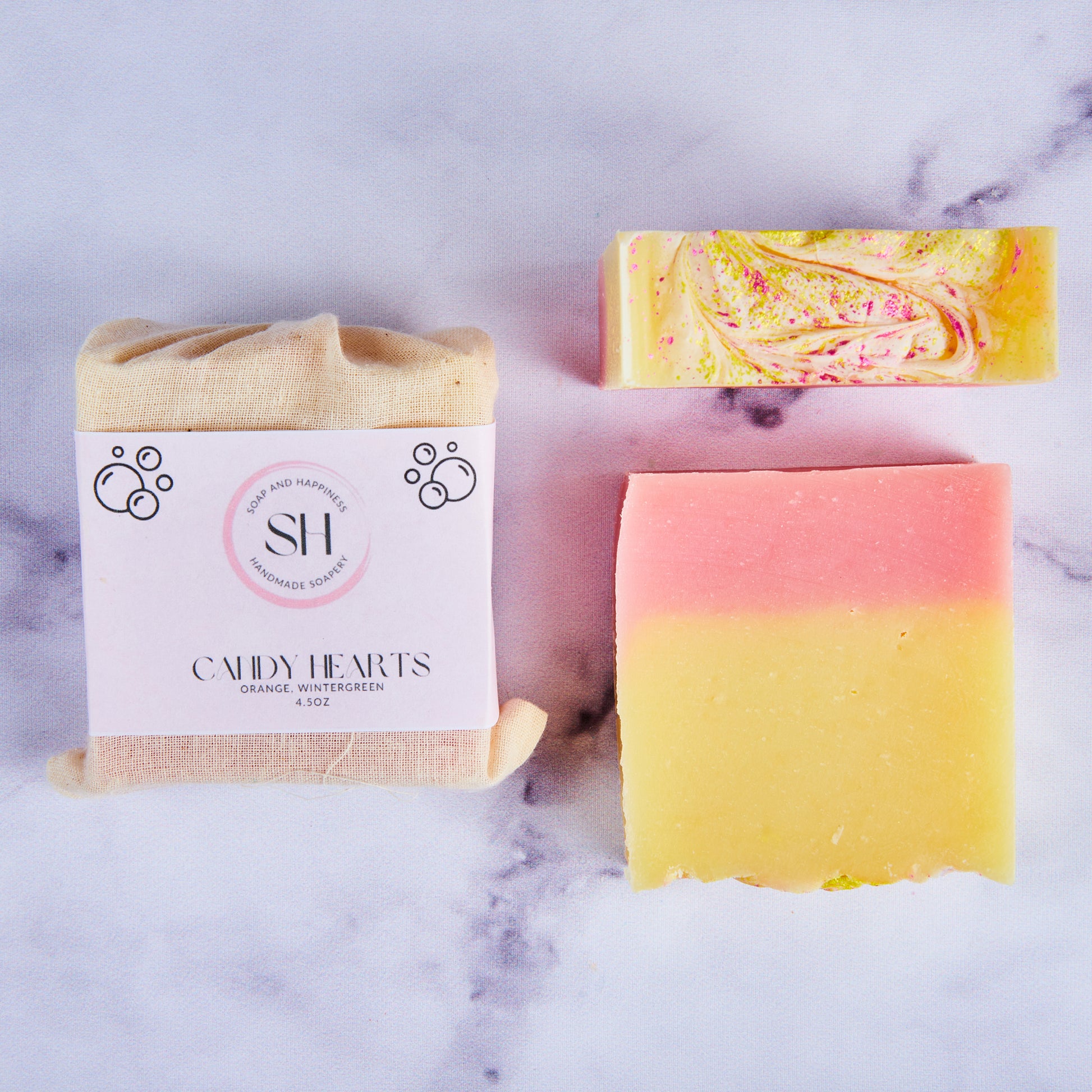This top-down photograph showcases three bars of Soap and Happiness (SH) handmade soap arranged artistically on a white and grey marble countertop, likely designed for an Instagram post or a small business webpage. The central soap bar, wrapped in a fabric and labeled "Candy Hearts - Orange, Wintergreen 4.5 ounces," features the SH brand logo, a pink bubble with bubbles embellishing the corners. On the right, one unwrapped bar stands on its edge, revealing intricate pink and purple swirls embedded within its yellow base layer, while another bar lies flat, presenting a uniform layer of pink on top and yellow below. The detailed visual composition highlights the artisanal quality and aesthetic appeal of the Candy Hearts soap, with its inviting scent and unique, artistic design.